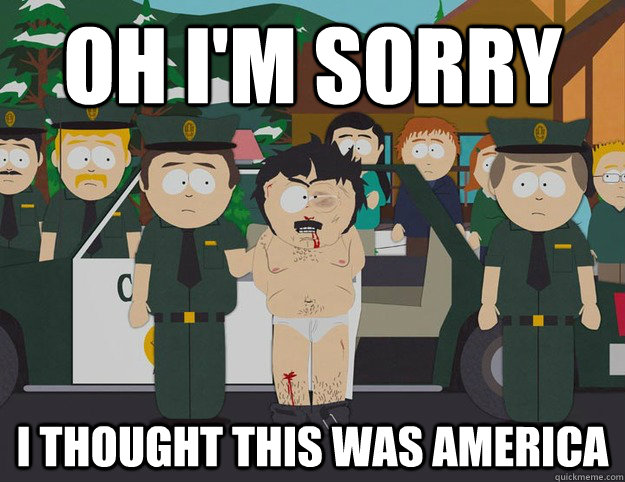A meme image features a muscular, bald Caucasian man lying on a bed, supported by his arms, with his legs presumably hidden under a red, gray, white, and black camo-patterned blanket. The man is nearly nude, sporting only a jockstrap or chaps, and he appears to be humping a pillow situated beneath him. He has a gray beard and mustache, short-trimmed facial hair, a tattoo on his right shoulder, and a noticeably hairy chest. Behind him, there are black and white striped pillows, possibly leather, and a dark wood headboard is visible against a gray wall. The room also contains white electrical outlets on either side of the bed. The meme features bold white impact font text at the bottom, outlined in black, that reads, "H-A-I."